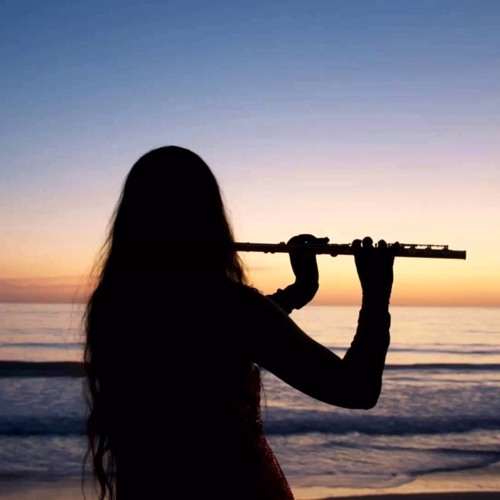In the image, a silhouetted woman with very long hair stands on the shore, facing the ocean as she plays a flute. The photo is taken from behind, revealing her extended arms holding the instrument to the right. The tranquil sea in front of her shows small waves gently crashing onto the beach, illuminated by the setting sun. The sky transitions from deep blues at the top to vibrant oranges and yellows near the horizon, blending beautifully as the sun casts elongated shadows, painting the water with dark blue and black highlights. This serene scene captures the peaceful moment just after sunset, with the woman immersed in her music against the backdrop of a slowly darkening sky.